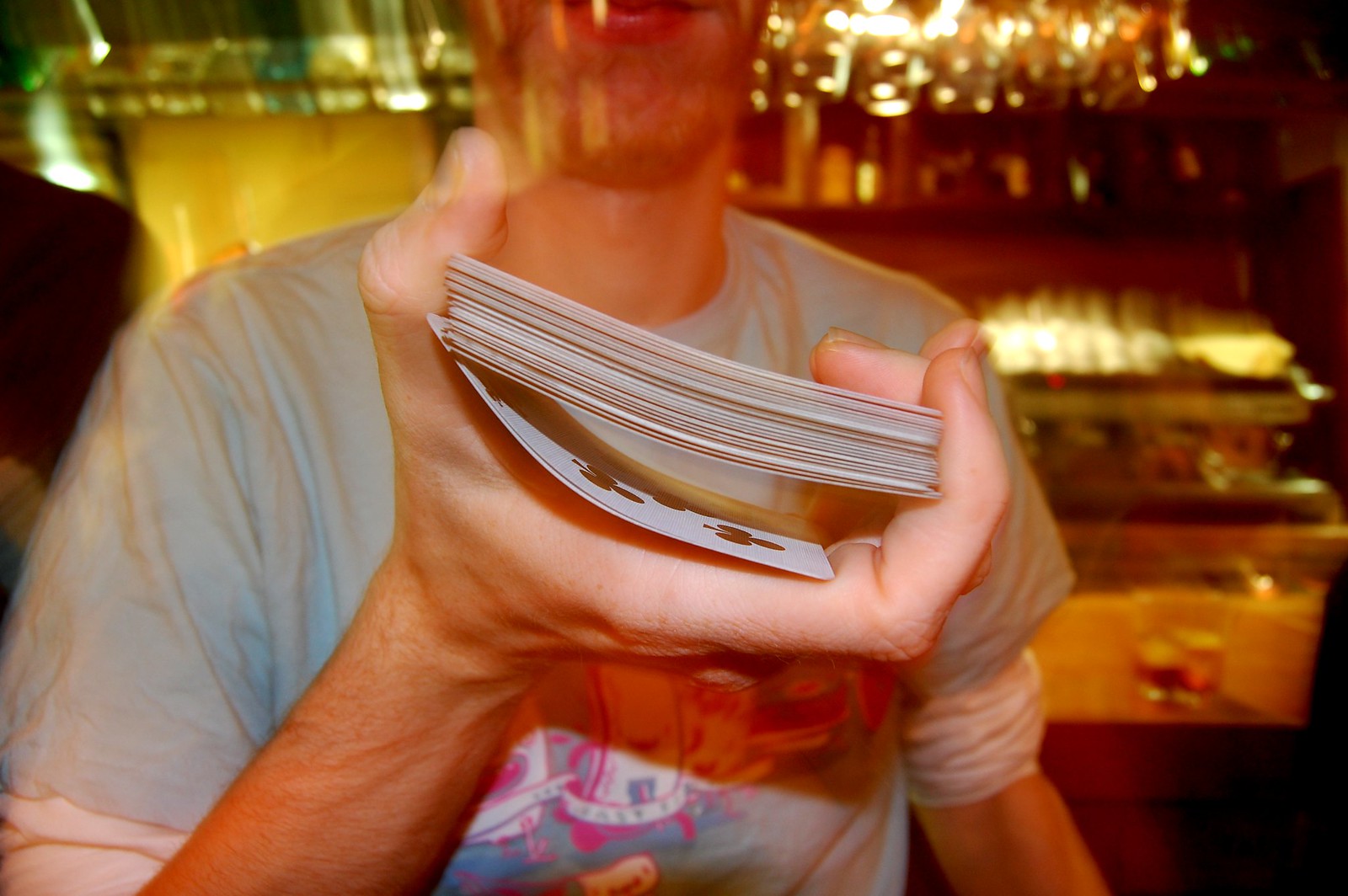A man, dressed in a gray shirt over a white long-sleeve inner shirt, stands in a dimly lit bar setting. The gray shirt features an animated image, though the design is partially obscured by his right hand. He holds a deck of cards, with the second to last card appearing to be the Eight of Clubs. The background is softly illuminated by yellow lighting, casting a warm glow over the scene. Behind the man, the silhouettes of wine glasses are faintly visible, hinting at the bar ambiance. On the right side of the image, two half-filled glasses of wine rest on the bar counter. It seems the man is preparing to perform a magic trick, possibly involving the deck of cards in his hand.